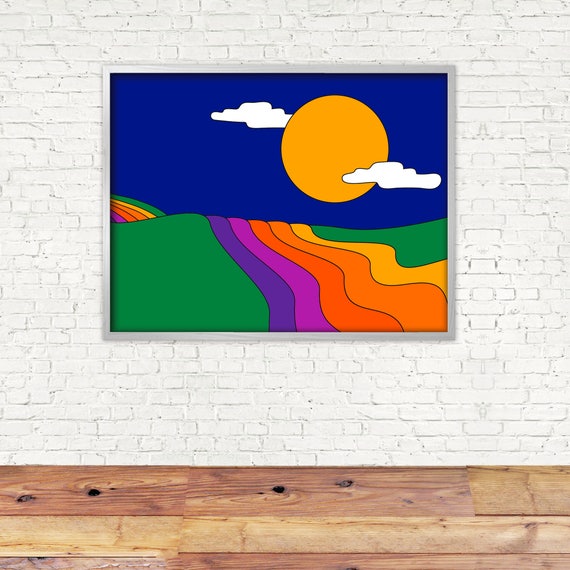This is a photograph capturing a vibrant piece of artwork mounted on a white subway brick wall. The lower portion of the wall features wide wood paneling in shades of dark and light browns. The artwork, enclosed in what appears to be a silver aluminum frame, showcases a colorful, animated scene. Dominating the scene is a large, golden sun set against a dark blue sky, flanked by two white clouds and a third partially obscured by the sun. Below the sky, a lush green field stretches out, traversed by a whimsical, wavy path resembling a rainbow. This path displays a captivating gradient of colors, including rich purples, varying shades of oranges, and yellows. The artwork's brilliant hues and dynamic composition create a striking contrast against the subdued tones of the brick and wood wall.